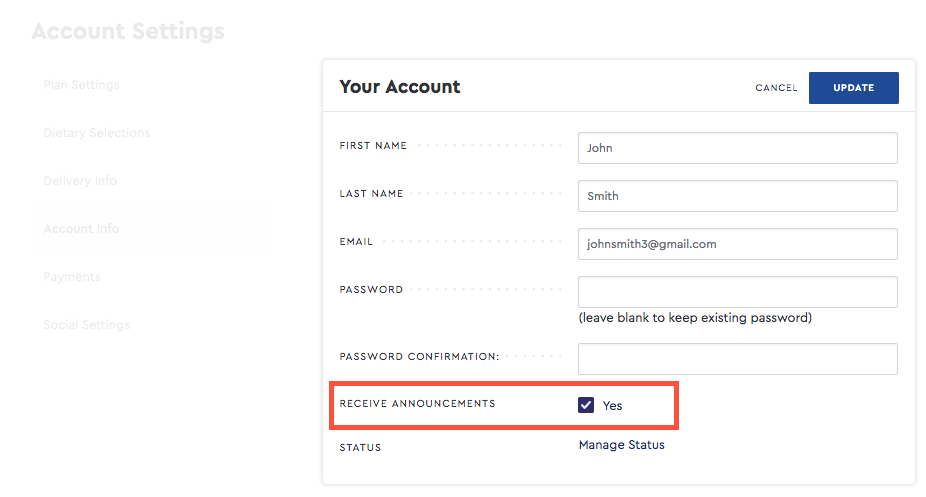The image depicts a user interface for account settings. On the far left, in very light text, the menu options include "Plan Settings," "Dietary Selections," "Delivery Info," "Account Info," "Payments," and "Social Settings." To the right in bold black letters, it prominently displays "Your Account" with options to cancel or update the account.

Below this, there are editable fields for personal information:
- "First Name:" followed by a long rectangular input box containing the name "John."
- "Last Name:" with an adjacent rectangular box containing the name "Smith."
- "Email:" to the right of this, the text "johnsmith3@gmail.com" is displayed.

For password management:
- "Password:" followed by an empty rectangular input box with a note in parentheses stating, "leave blank to keep existing password."
- "Password Confirmation:" includes an adjacent empty input box.

The section for communication preferences has "Receive Announcements" highlighted in red, with a checkbox next to the word "Yes," which is checked. Underneath this, there are options for managing user status, indicated by the words "Status" and "Manage Status."